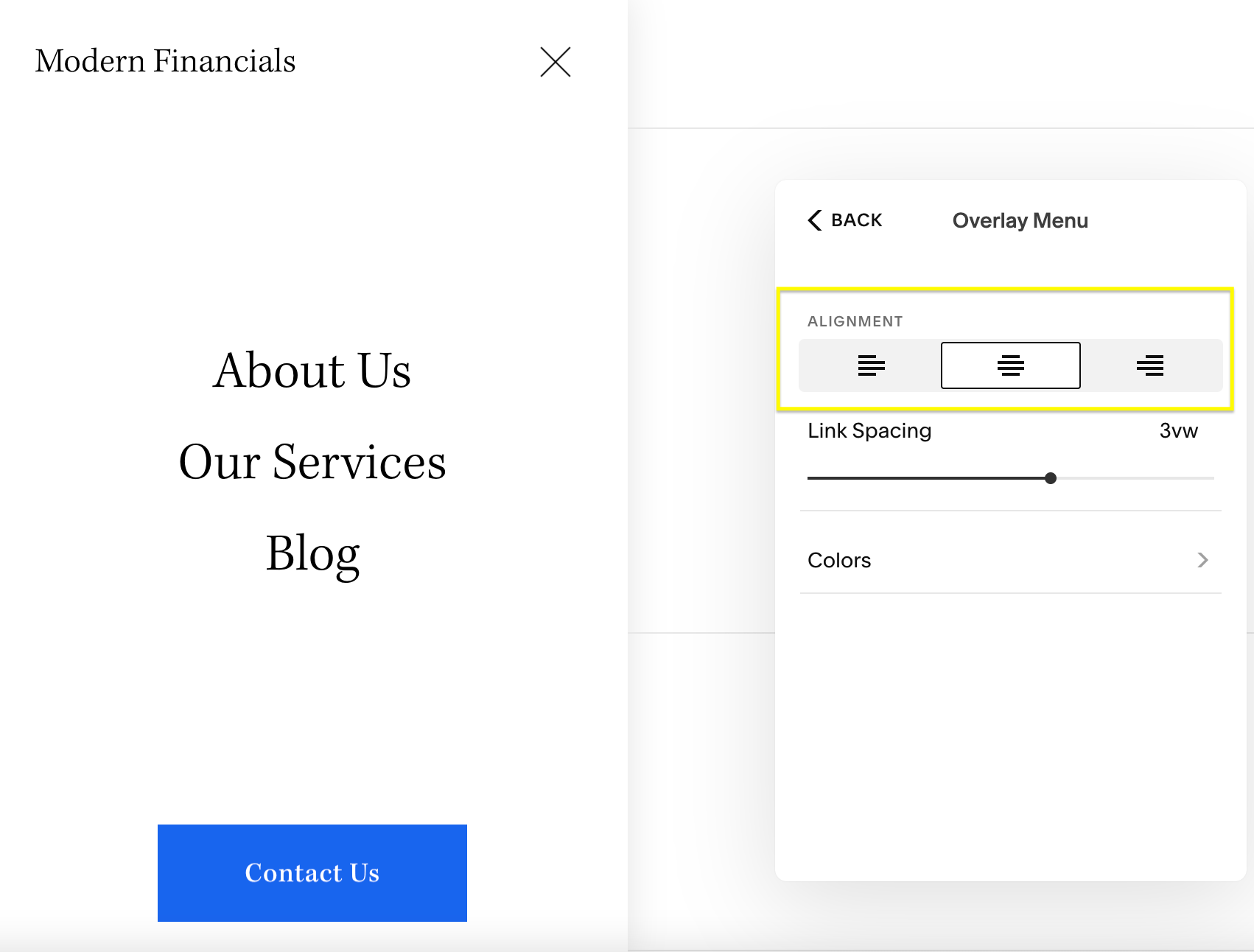The image depicted is a screenshot from a computer screen, featuring a user interface with a clean, modern design. The left side of the screen showcases a tall, rectangular panel with a predominantly white background. At the top of this panel, the text "Modern Financials" is prominently displayed in black print, accompanied by a close (x) icon. 

Beneath this heading, several menu options are listed including "About Us," "Our Services," and "Blog." Lower down, there is a blue rectangular box containing the text "Contact Us."

The right side of the screen presents a whitish-gray rectangular area. Below this section is an interactive button labeled "Back," complete with an arrow icon for navigation. This area also features an overlay menu, outlined by a yellow rectangular line that encompasses the alignment settings.

Within this yellow-lined area, the alignment settings offer multiple options. The middle alignment option has been selected, centering the content within the designated space. Additional settings for link spacing and colors are visible, indicating further customization options for the user interface.